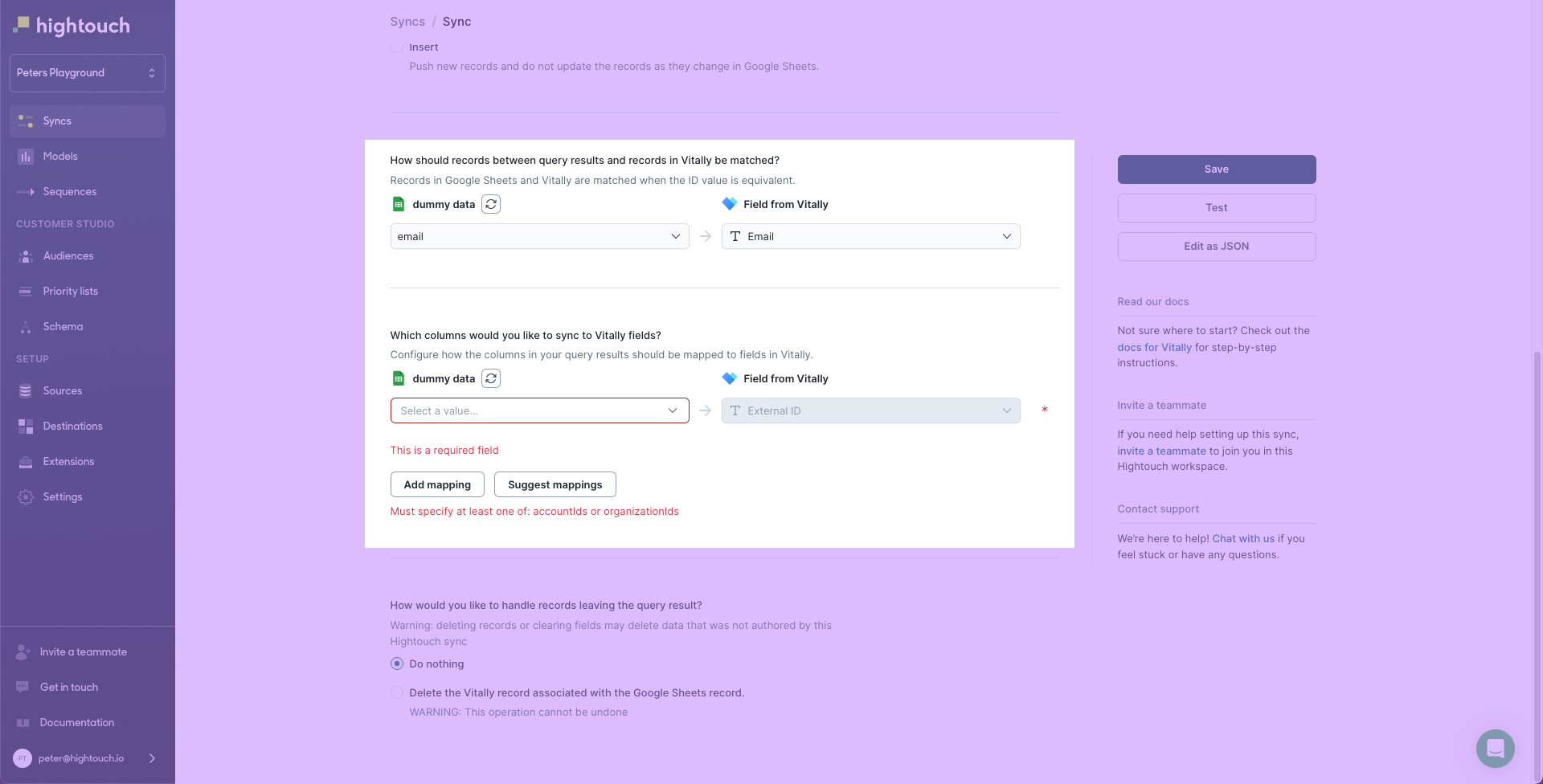The image features an intensive pink filter overlay across the entire composition. On the left side, a vertical bar is prominently visible with the words "high touch" written on it. Underneath this bar, there is a search bar followed by a menu displaying various categories, though the text is small and difficult to read due to the pink overlay.

In the center, a white pop-up box is noticeably present. This box contains several text fields and additional text above, although much of this text is illegible due to the image being stretched and resized. Behind the white pop-up box, more lines of text are visible, continuing downward, but are also hard to decipher.

On the right side, there are multiple buttons, including a highlighted blue button and two grayed-out buttons with additional text beneath them, which again is too small to be readable. Additionally, in the bottom right corner, a blue circular button is noticeable, featuring an unclear white icon that looks somewhat like a page, though the details are obscured by the pervasive pink filter.

Overall, the image is dominated by a pink background that affects the clarity and readability of various elements, including categories, text fields, and buttons.